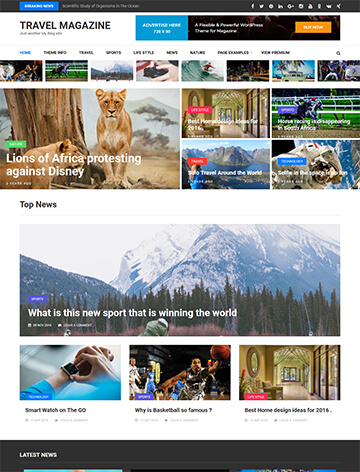This image appears to be a webpage from "Travel Magazine." In the top left corner, the title "Travel Magazine" is prominently displayed. On the top right, there is a series of small white icons including a speaker (indicating muted sound) and various social media logos such as Facebook, Twitter, LinkedIn, Gmail, and Steam.

Centrally, the main section features a notable image of two lions or lionesses with a caption beneath it that reads, "Lions of Africa Protesting Against Disney." To the right, the layout consists of four smaller, separate boxes, each containing a different picture: the top left box shows a home, the top right features a horse race, the bottom left presents an ocean view, and the bottom right depicts an astronaut.

Further down, on the middle left of the image, the heading "Top News" is displayed in black text. Adjacent to this, there's a large rectangular box with the headline, "What is this new sport that is winning the world?" The background of this section is an expansive snowy mountain range with a green forest stretching horizontally across the bottom.